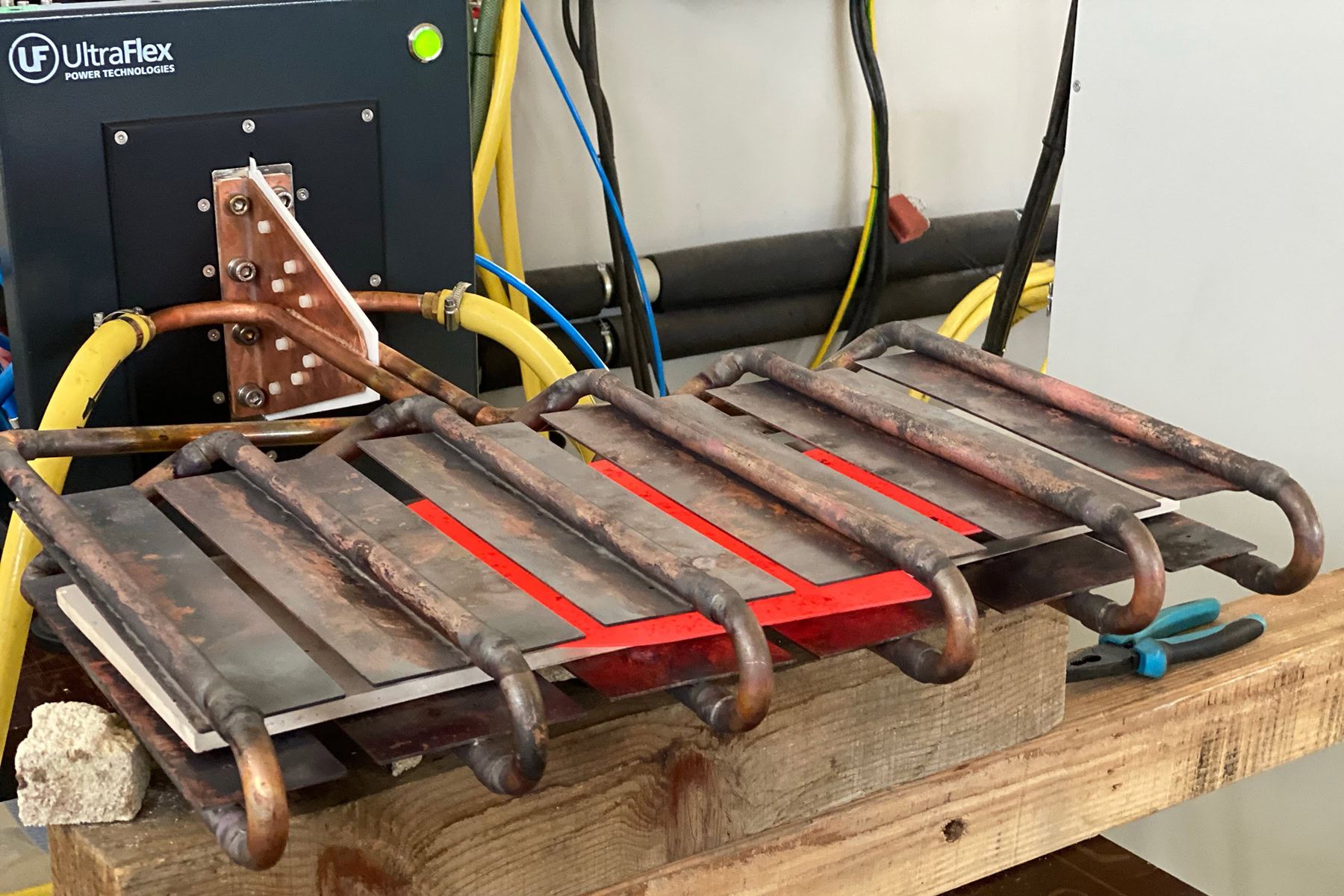This image captures a close-up shot of an intricate machinery setup on a wooden workbench. Central to the scene is a large metal apparatus comprising copper tubes, some of which are rusted, connected to yellow rubber pipes. The copper tubing loops in a circular fashion around metal plates and extends toward a black box affixed to a white wall, which also has black tubes emerging from its right side. The machinery, a mix of copper and steel elements, is partially supported by two wooden studs. On the left wooden stud, there is a white square stone, while the right stud holds a pair of black pliers with blue handles. An Ultraflex Power Technologies logo featuring "UF" is visible in the upper left corner, suggesting the machinery's branding. The overall scene, cluttered yet detailed, indicates an ongoing repair or assembly work on this complex device.